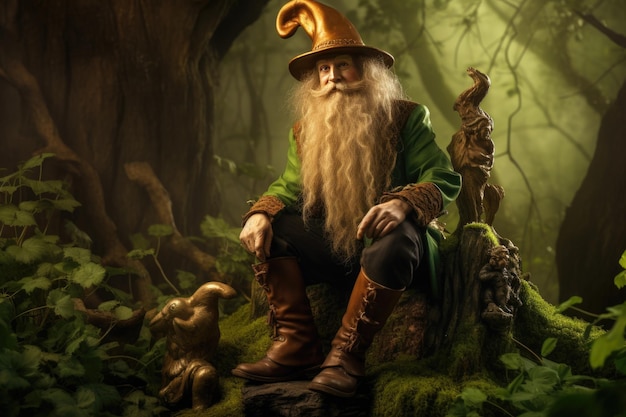This highly detailed, potentially AI-generated or digitally created image depicts a fantasy character prominently centered. The character, evocative of elves, dwarfs, or wizards from stories like "Lord of the Rings," has a striking appearance with long, wavy white hair, a flowing beard, and a large, pointed white mustache. He dons a gold-colored, whimsically curved hat that resembles a wizard's hat, along with a long-sleeved green shirt with gold cuffs, black trousers, and brown leather boots.

Seated on an ornamental tree stump draped with moss and foliage, the character has his hands resting on his knees, seemingly deep in thought with eyes staring into the distance. In front of his boots lies a carved wooden bird. The background is suffused with a light green hue, suggesting sunlight filtering through dense forest foliage, augmented by a foggy ambiance. To his left is a massive tree, entwined with vines and branches, while to his right stands a statue of a woman with a large headdress. His surroundings hint at a deep, magical forest setting, filled with an air of mystery and enchantment.